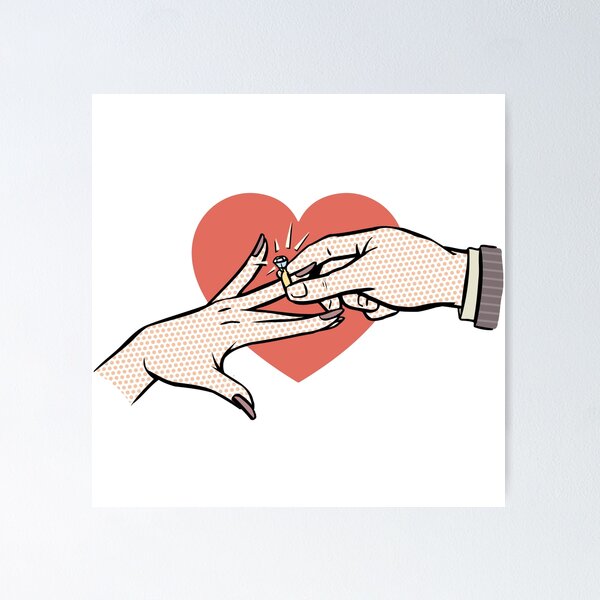The image depicts a whimsical, square poster or print with a white background framed by a blue border. At the center, a charming engagement scene is illustrated in a cartoon style reminiscent of old comic books, using a distinctive dot pattern for shading. From the left, a woman's hand with light purple, long, polished nails extends towards a man's hand on the right. The man's hand, emerging from a gray, pinstriped suit sleeve with a white shirt peeking out, delicately places a sizable gold diamond ring on the woman's ring finger. A vibrant red heart frames the point where their hands meet, symbolizing true love. Both hands are composed of tiny pink dots, adding to the nostalgic comic book feel of the image.